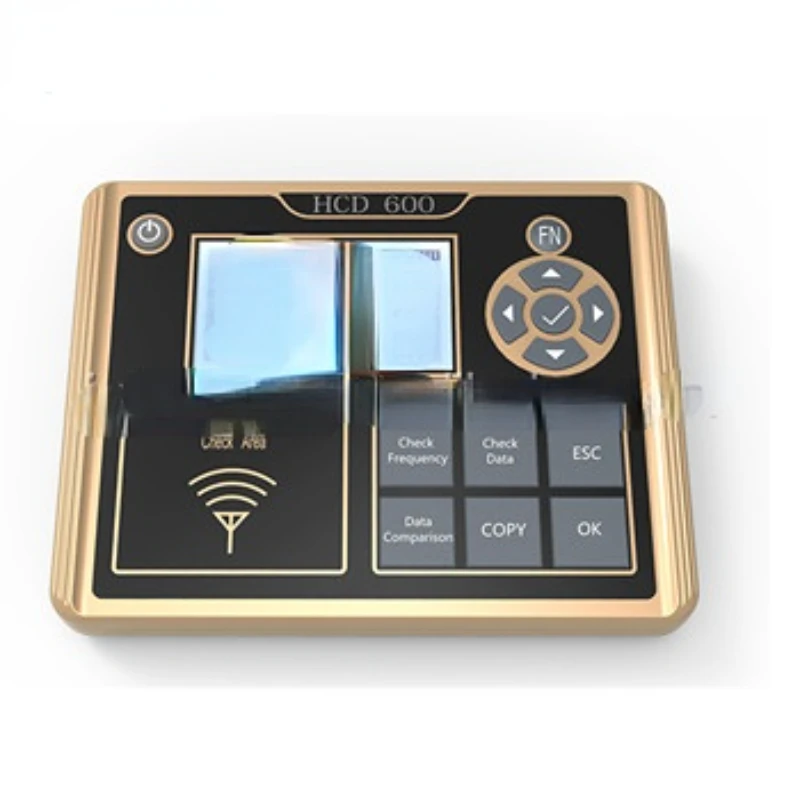This photograph showcases a sleek, square electronic device, predominantly black with a pale gold trim, resting on a white background. At the center of the device, it is labeled "HCD 600." The upper left corner features a soft power button, while the upper right corner consists of a directional pad with arrows pointing up, down, left, and right, and a check mark in the center. Just above this directional pad is a circular soft button marked "FN." Below the directional pad on the bottom right, there are six rectangular buttons arranged in a 2x3 grid, labeled "Check Frequency," "Check Data," "ESC," "Data Comparison," "Copy," and "OK." In the bottom left corner, there is a Wi-Fi symbol icon with the words "Check Area" above it. Above this section sits a light blue square LCD screen. The device, crafted with a metal casing, has a slightly fuzzy and distorted appearance in some areas. The exact function of the device remains ambiguous, though it resembles a remote control.